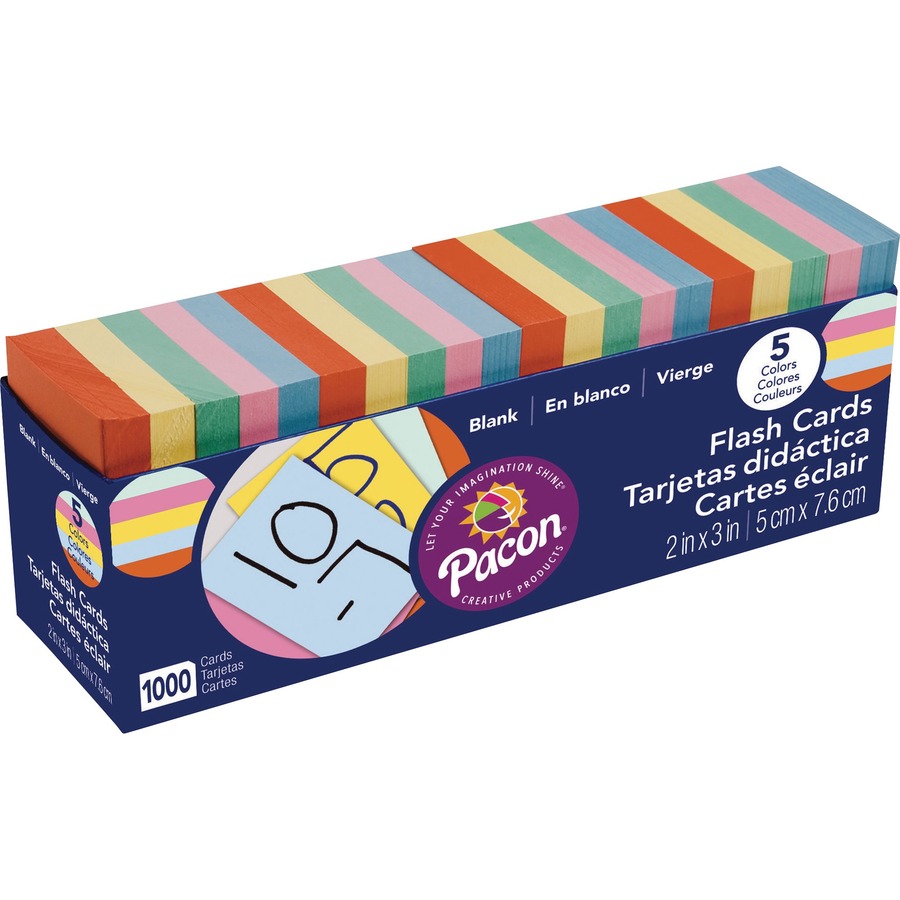The image depicts a long rectangular box of flashcards without a lid, displaying a total of 1,000 cards in an organized and colorful fashion. The cards are neatly arranged in repeated sets of five colors: orange, yellow, green, pink, and blue. The arrangement continues throughout the box. The front of the dark blue box features a variety of multilingual text and illustrations. Prominently, the bright round purple logo of "PACON" is accompanied by the slogan "Let your imagination shine" and "Creative Products." Adjacent to this logo, another circle illustrates a blue flashcard with a math equation (10-7), and a yellow flashcard with the number 5 peeking from behind it. The packaging also details the dimensions of the cards as 2 inches by 3 inches or 5 centimeters by 7.6 centimeters. The words "flashcards," "tarjetas didácticas," and "cartes éclair" are printed in three languages: English, Spanish, and French, along with other descriptors like "blank" (en blanco, vierge) and "five colors" (colores, couleurs). The back and sides of the box repeat these multilingual details and include additional illustrations of the flashcards. This visual suggests that the image might be used for advertising or web display due to its clean and straightforward presentation against a white background.